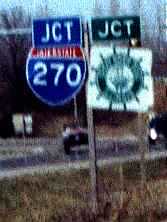This is a small, color photograph depicting a somewhat blurred roadside scene with poor resolution. On the left side of the image, there are several road signs. One prominent sign is blue and red with white writing, displaying "JC1" above "270." Adjacent to it is a green sign at the top with white letters, also indicating "JC1." Beneath that, a white sign showcases a green object resembling either a sun or a flower, characterized by a round edge with spikes. Within this green object, there is a white circle containing an unreadable green logo. Below the signs, there is a stretch of grass. The background reveals a road with a vehicle in motion and a line of trees extending beyond the signs. More road signs can be seen in the distance on the left side, and the scene is capped by a clear blue sky.